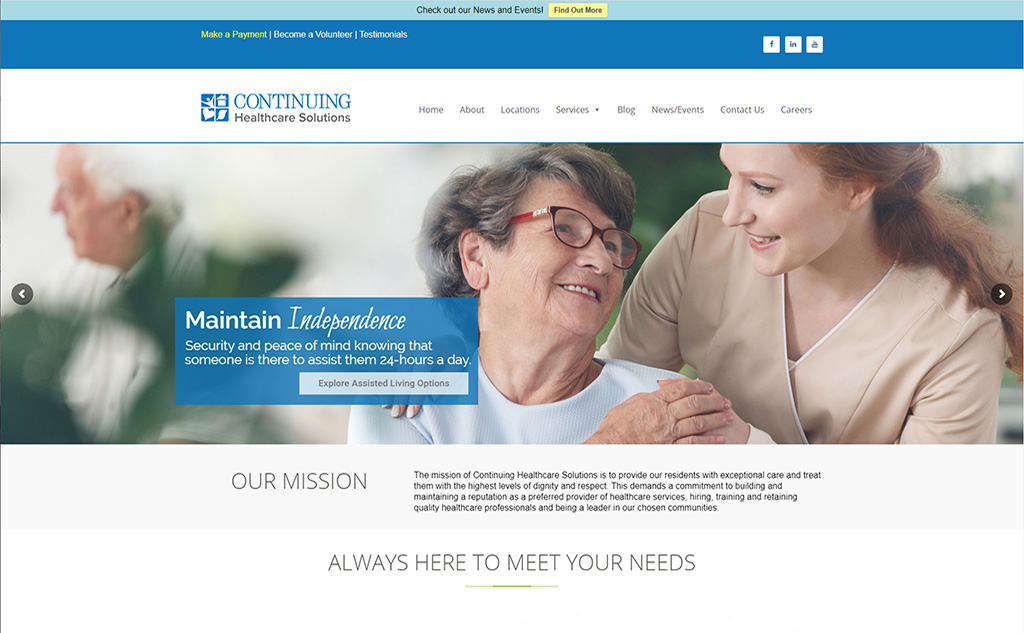This screenshot captures the homepage of the Continuing Healthcare Solutions website. The website name, “Continuing Healthcare Solutions,” is prominently displayed in the upper left corner, next to their distinctive logo featuring four blue squares, each containing a unique symbol: an acorn, a leaf, a heart, and a figure with arms outstretched.

At the very top of the page, a blue banner invites visitors to “Check out our news and events,” with a yellow “Find out more” button adjacent to it. This banner also hosts links for “Make a Payment,” “Become a Volunteer,” and “Testimonials.” To the right, there are small square icons linking to Facebook, LinkedIn, and another social media platform.

Central to the webpage, there is a heartwarming image of an older woman and a younger woman who appears to be either a nurse or a family member, engaged in a compassionate interaction. The older woman’s setting suggests she is in a healthcare facility. Overlaid on this image is a comforting message: "Maintain Independence, Security, and Peace of Mind, knowing that someone is there to assist them 24 hours a day." Below this message, a prominent button reads, “Explore Assisted Living Options,” emphasizing the website’s commitment to meeting the needs of their residents.